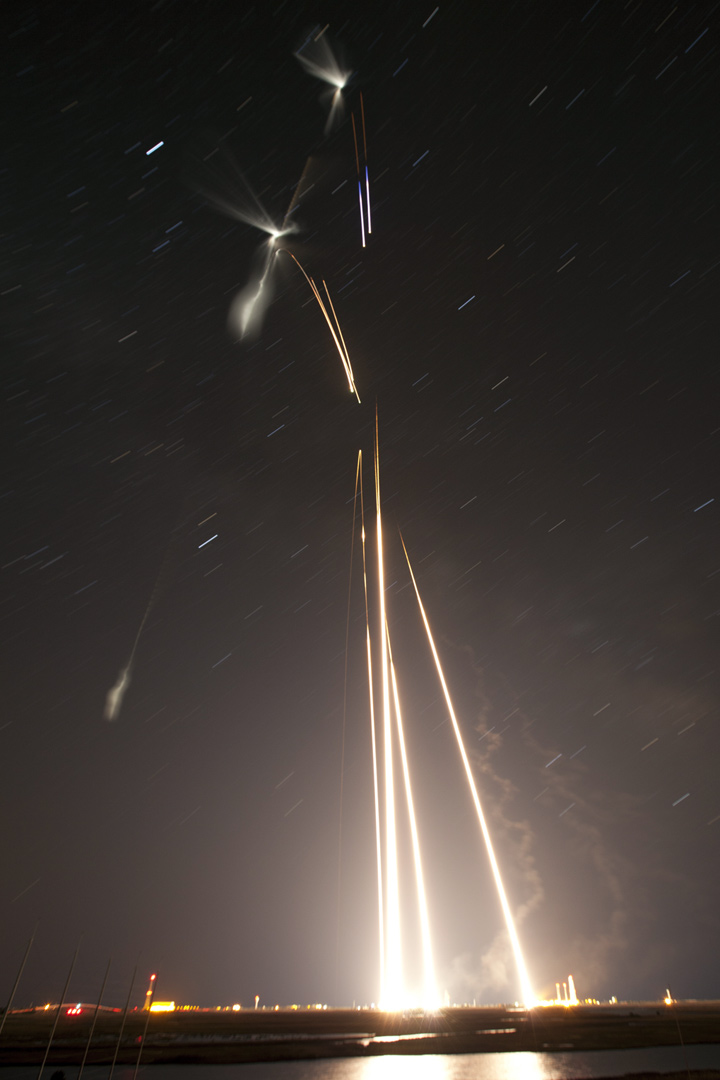The photo captures a nighttime scene with a dark sky that gradually lightens towards the horizon, emphasizing the backdrop of an indiscernible cityscape with faint neon lights. In the foreground, there is a body of water which reflects bright, thick streams of light. Four prominent beams of light emanate from the ground, where small buildings are barely visible. These beams widen and brighten towards their base. As these beams ascend, they give way to numerous thinner strands of light, falling and leaving trails behind. The scene is further accented by two zigzag waves of smoke on the right side, and small dashes of light streaking from the top right corner to the left, almost resembling falling stars. The ambiguity of the situation, with elements resembling fireworks, a missile launch, or a light show, adds a sense of mystery and dynamism to the otherwise stark and empty landscape.